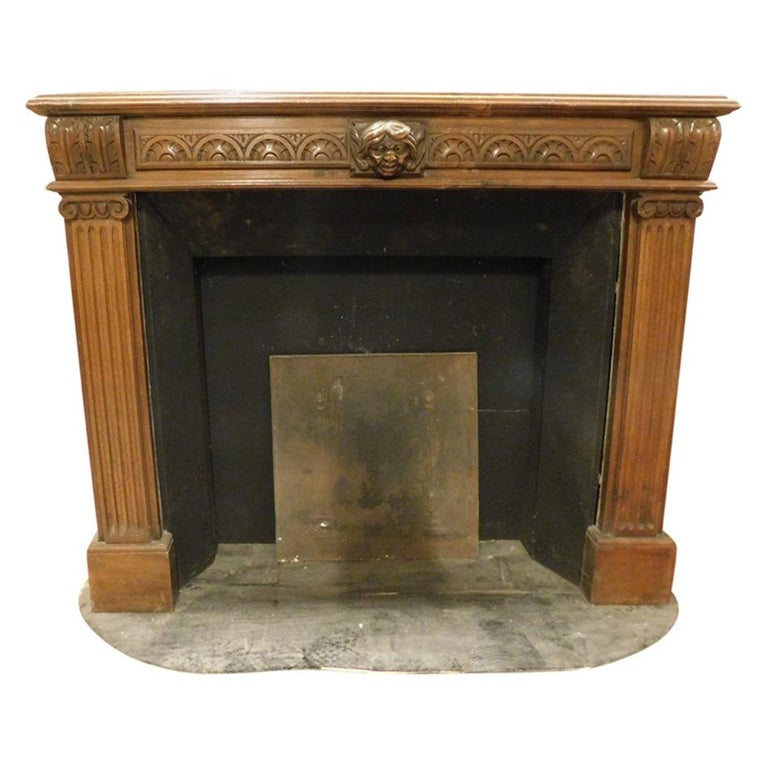This detailed photograph showcases an old, elaborately designed fireplace that has been visually isolated against a stark white background, suggesting it has been either photoshopped or meticulously cut out from a larger image. The fireplace is flanked by two intricately carved pillars that resemble wood but are likely crafted from a molded material and painted brown. The top, serving as the mantel, appears to be made of heavy-duty wood, possibly mahogany, featuring a row of carved semicircles and a prominent face at the center. This unsettling face, with its goblin-like features and metallic sheen, adds a peculiar and almost demonic touch to the piece. The interior of the fireplace is stark black, with remnants of ash and soot visible on the concrete floor, indicating it was used at some point. At the back, a charred metal plate stands, further adding to the weathered and historical ambiance. The overall composition, with its mix of materials and detailed carvings, evokes a sense of age and mystery, making it a striking subject of interest.